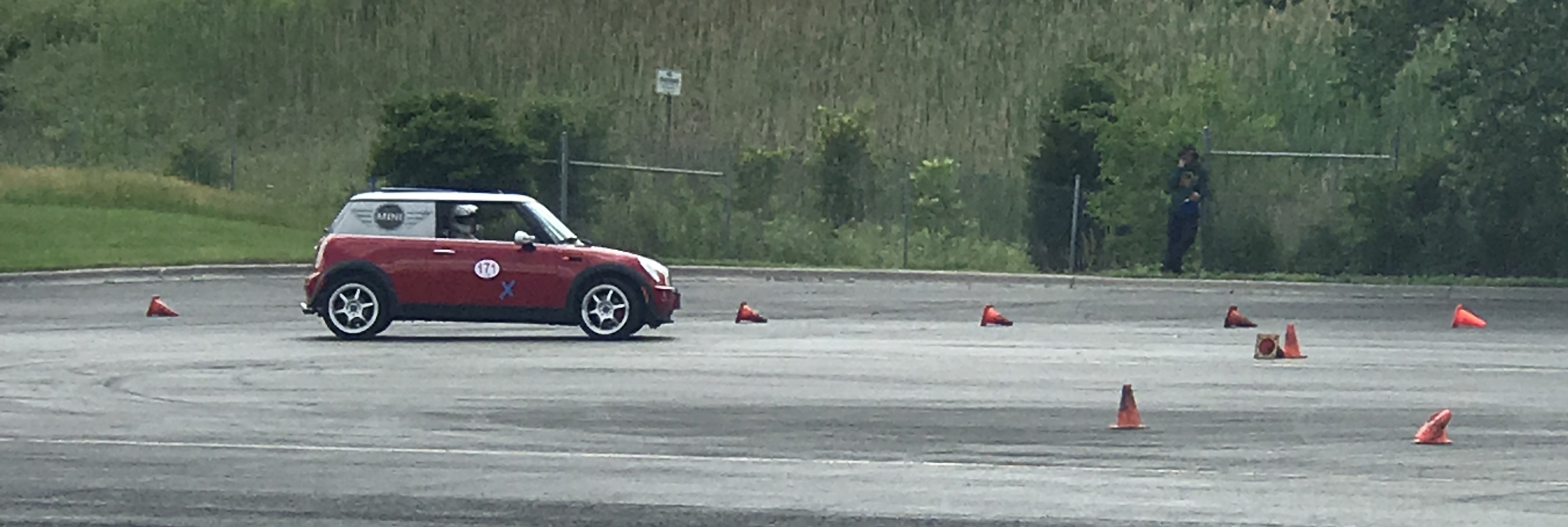The image depicts a long, rectangular obstacle course designed to test a car's handling on a cement parking lot. The upper half of the image features a green hill and a high chain-link fence with tall shrubs against it. The lower half showcases a sleek, paved area. A red Mini Cooper with black wheels, silver hubcaps, and a white top dominates the left side of the image, moving toward the right. The car sports a white circle on its door marked with the number 171 and a blue 'X'. The driver, donning a white helmet, sits on the right side, indicating a British setup. Scattered throughout the lot are various small orange cones—nearly all of them knocked over, except for three. In the background, a person dressed in black leans against the fence, seemingly using a cellphone. Additionally, a small white sign on a metal pole stands at the edge of the lot.